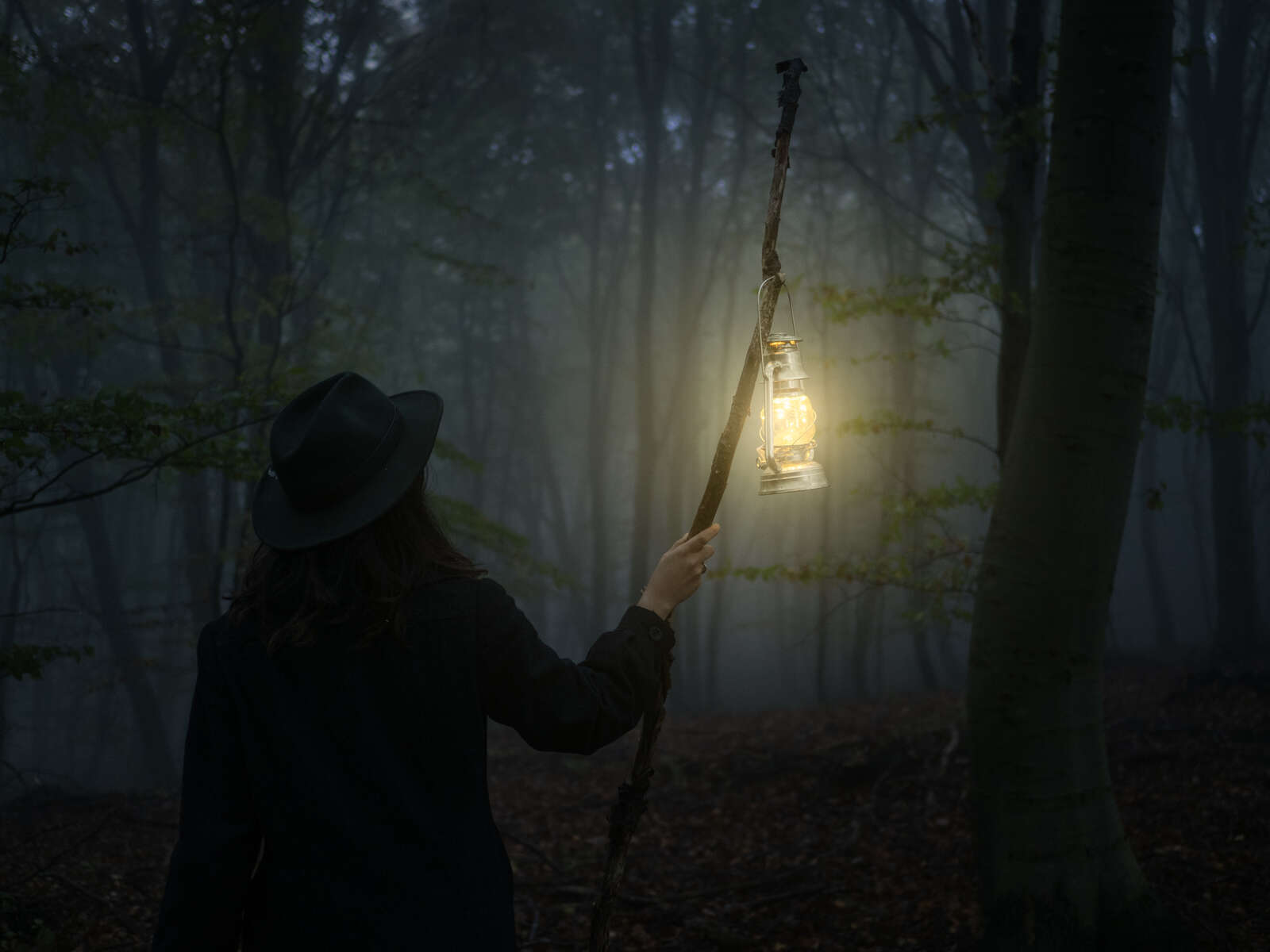The photograph features a solitary woman standing in a dimly lit, misty forest at night. She holds a long wooden stick in her right hand, adorned with a bright silver lantern, which casts a warm, yellow glow, softly illuminating her path through the fog. She stands to the front left of the image, dressed in dark clothing: a dark blue or black jacket, long brown hair cascading down her back, and a black brimmed hat that resembles a trilby fedora. The largest tree, roughly 12 inches in diameter, stands prominently at the right front of the image, with numerous smaller trees receding into the background shrouded in mist. The forest floor is scattered with brown leaves, fallen twigs, and logs, creating a textured carpet under her feet. While most of the sky is obscured by the canopy, faint patches of light peek through the treetops. The overall atmosphere of the scene is eerie and mysterious, bathed in the lantern's glow and the ethereal light filtering through the trees.